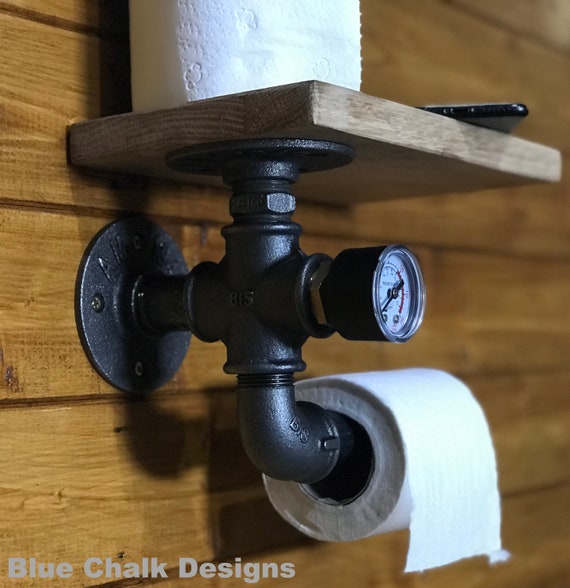The image depicts a creatively designed toilet paper holder and shelf, crafted from black piping and wood, set against a plain brown wooden wall. The structure features a black circular metal base screwed into the wall, from which a pipe extends vertically, connecting to a four-point cross joint. One arm of the joint leads downwards to an elbow joint that holds a horizontally placed white roll of toilet paper. Another arm of the cross joint supports a white-faced pressure gauge with a black needle, adding an industrial touch to the holder. Above the cross joint, an oak-colored wooden shelf is mounted, held up by the vertical pipe. This shelf houses an additional roll of toilet paper and a corner of a cell phone is visible resting on it. Shadows cast by the lighting in the room add depth to the scene. In the lower left-hand corner of the image, the text "blue chalk designs" is clearly displayed, indicating the creator or design inspiration.